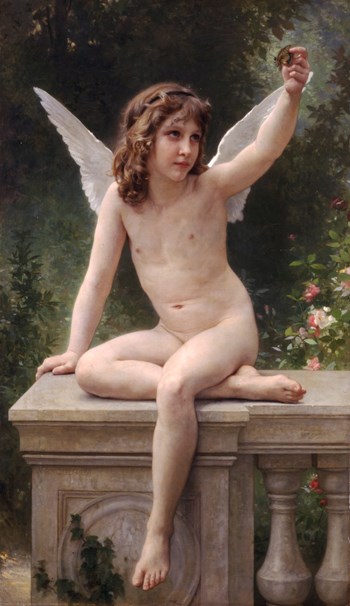This detailed painting captures a realistic image of a young, nude angelic girl, sitting gracefully on a stone wall designed in an ancient Greek architectural style, adorned with pillars. Her delicate white wings, indicative of her angelic nature, extend from her back. With shoulder-length curly brown hair held back by a black hairband, she gazes intently at a butterfly which she gently holds between her index finger and thumb, her head turned to observe it. Her left leg rests over her right, and she supports herself with her right hand on the stone surface. The background reveals a lush, green forest with light filtering through, interspersed with pink and white flowers, and green leaves below her. The setting is bathed in daylight, adding to the serene and ethereal quality of the scene.